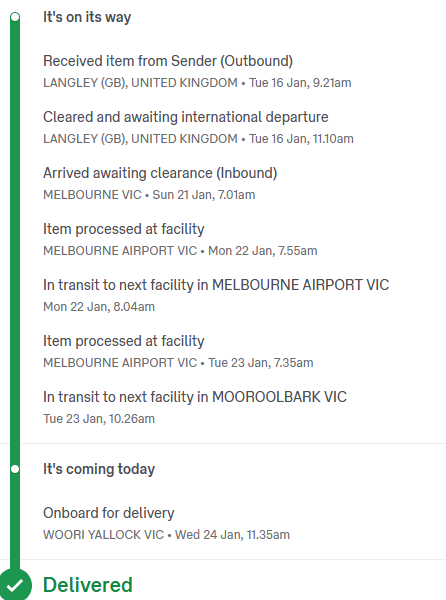This image is a screenshot of a delivery tracking webpage. At the top, the page summary indicates that a delivery is in progress. The central section prominently features a green checkmark on the bottom left, symbolizing successful delivery. A green progress bar originates from the top left and descends towards this checkmark, with two white dots along its path—one at the very top and one near the bottom—indicating key milestones.

On the right side, a detailed timeline of the parcel's journey is visible, enumerating various checkpoints and statuses. The first entry reads, "Received item from sender," specifying it is outbound, followed by the origin location. The next status is "Cleared and awaiting international departure," accompanied by the place, date, and time. 

Following this, the entry states, "Arrived and awaiting clearance inbound," again detailing the location, date, and time. The timeline continues with "Item processed at facility," followed by specific details of the location, date, and time. It then mentions "In transit to the next facility in Melbourne Airport, VIC," along with the corresponding date and time.

Further down, the image shows "Items processed at facility," with the location, date, and time, and once more marks "In transit to next facility in Morro Park, VIC," with date and time. At the very bottom, bold green text highlights that the item has been delivered, with the final entry recounting the delivery as "Coming today: outbound delivery," followed by the place, date, and time.